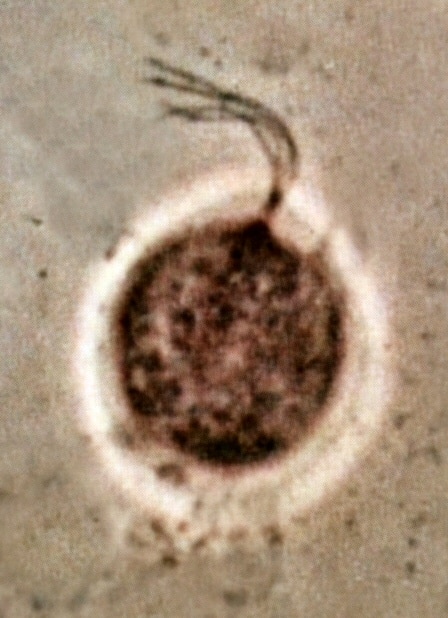The image shows a highly magnified, blurry object that appears to be a microscopic organism or cell against a light beige to grayish background. The background is unevenly speckled with dark brown or black spots, particularly dense in the bottom right corner. At the center of the image, there is a prominently round, flat, brownish object with an uneven, almost muddy texture. This central object is surrounded by a distinct white circle which appears layered, especially towards the front. Several dark, hair-like strands or tentacles extend from the top of the brownish circle, protruding through the white ring. The overall appearance of the object gives it a somewhat brain-like texture, suggesting it might be a biological specimen viewed under a microscope, potentially in a clinical or laboratory setting.